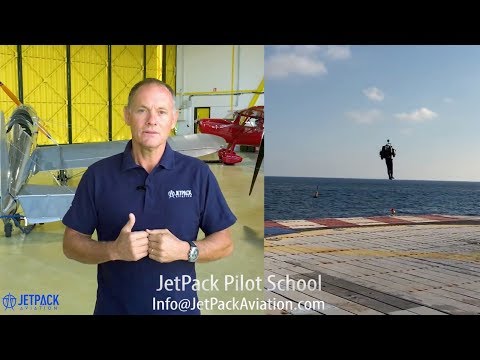In this image, we see an elderly man wearing a blue shirt emblazoned with the Jetpack Aviation logo. The image is split down the middle, with two distinct scenes. On the left side, the man stands inside a large hangar, identifiable by reflective marble floors and walls adorned with yellow and white piping. Behind him are two airplanes: a silver plane to his left and a red one partially visible in the background. His stance suggests he might be addressing an audience, with hands positioned as if giving a thumbs-up gesture, and he is wearing a wristwatch on his left hand.

On the right side of the image, a person is flying a jetpack above a platform situated in the ocean. The platform has a gray, brick-styled pattern and serves as a stark contrast to the clear, blue sky and the deep water. The image prominently features text that reads "Jetpack Pilot School Info at JetpackAviation.com" at the bottom left, reinforcing the promotional nature of the photograph.